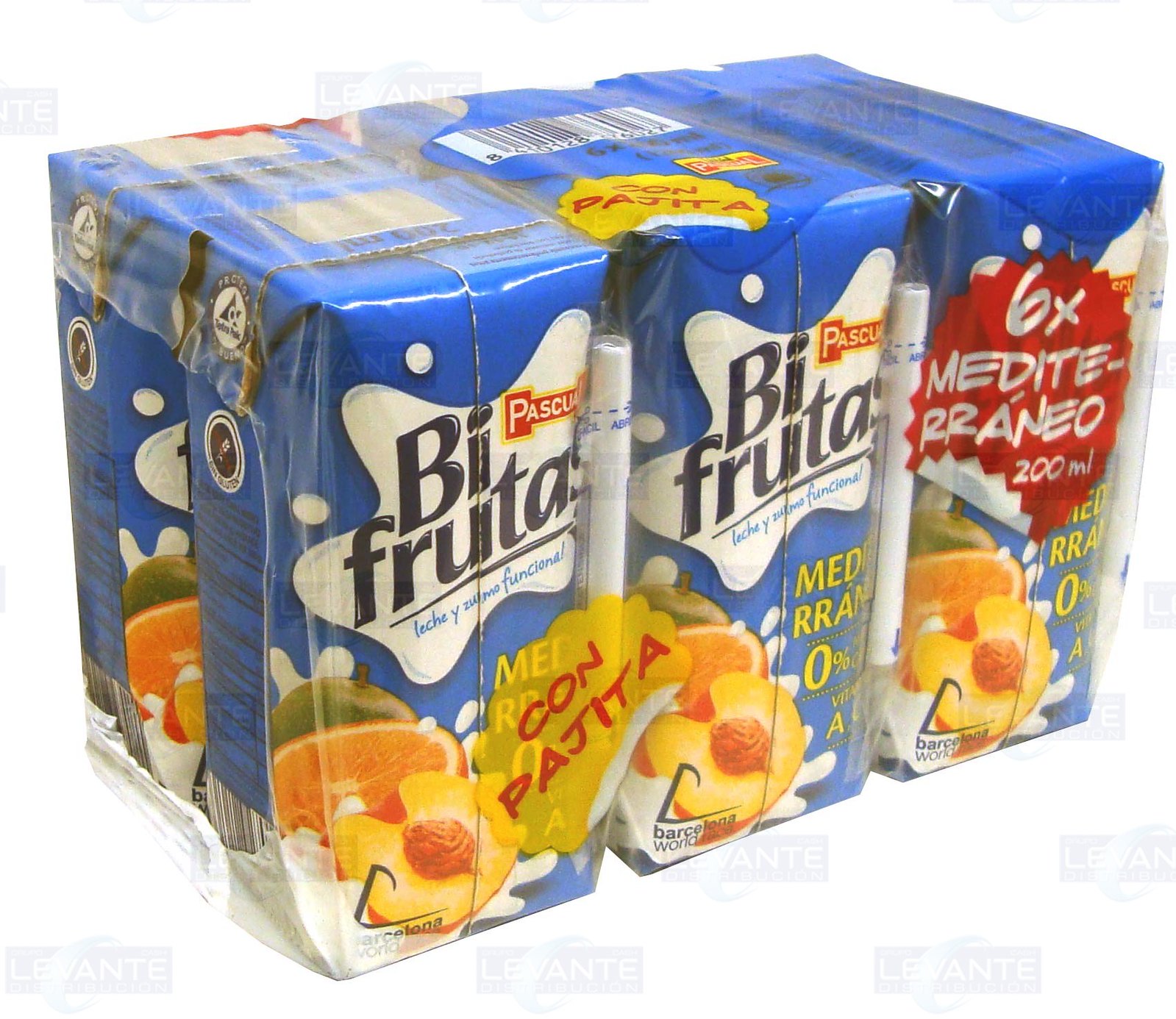This colour photograph depicts a six-pack of carton drinks, shrink-wrapped together, resembling an online grocery store product image. Each carton, predominantly dark blue, features its own straw attached on the front. The product appears to be foreign, as indicated by the red text "Con Pajita" in a yellow, cloud-shaped bubble on the front, which translates to "with straw" in Spanish. The brand name "Bifrutas" is displayed prominently within a white splash design, and above it, the phrase "leche y zumo funcional" indicates a blend of milk and juice.

The front of each carton shows a detailed cross-section of a peach, an orange behind it, and what seems to be a green apple in the background. The packaging also includes numerous labels such as "Mediteráneo," "cero por ciento" (zero percent), and "vitamina A", emphasizing health benefits. Additionally, there's a repeating, faded watermark logo, likely from the retailer, indicating "Levante."

The six-pack holds 200 milliliters per carton, as stated near the top, along with the description "six times Medite Raneo." The fruits and design suggest a refreshing, possibly Mediterranean-inspired beverage, aimed at a broad audience, possibly including children, given the convenience of the attached straws.